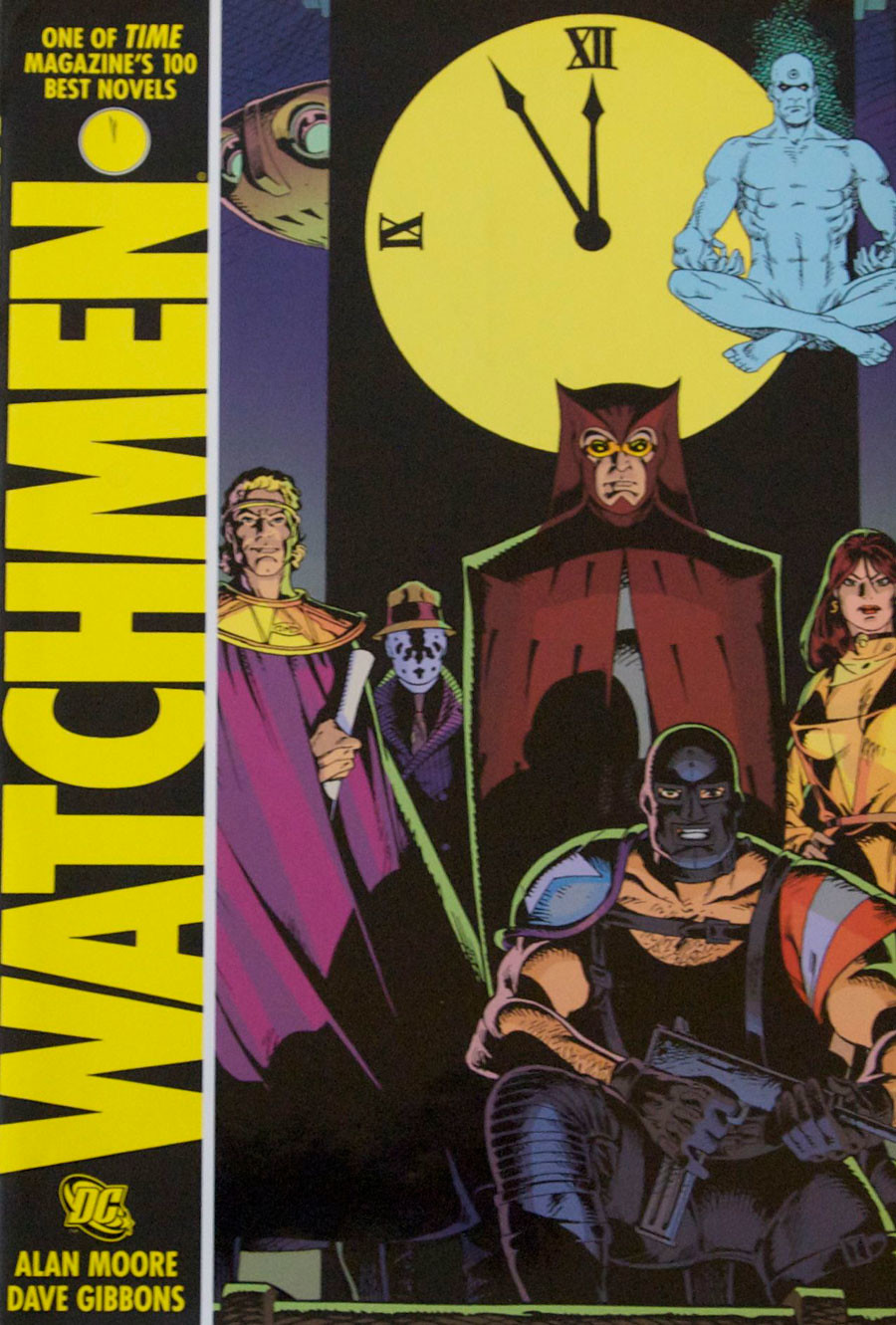The image appears to be the cover of the iconic comic book "Watchmen". Dominating the left side, there's a long vertical yellow rectangle with the text "One of Time magazine's 100 best novels" at the top. Below this, the title "Watchmen" is prominently displayed in large yellow letters turned vertically. Beneath the title, in the same yellow lettering, are the names "Alan Moore" and "Dave Gibbons" along with the DC Comics logo. The background transitions into a deep purple on the right side, featuring a large black rectangle with a yellow clock face exhibiting Roman numerals. The clock shows approximately 11:55, suggesting an imminent event. To the right of the clock, a muscular, bald blue man sits cross-legged, exuding a sense of calm. Below the clock, several characters are grouped together. One character, donning a black mask and wielding a pistol, has shields on his shoulders. Nearby, another person is dressed in a purple robe, golden tunic, and crown. Additionally, a woman with brown hair is depicted wearing a yellow and black blouse. These characters, with their distinct appearances and poses, collectively underscore the dramatic and intricate nature of the "Watchmen" universe.